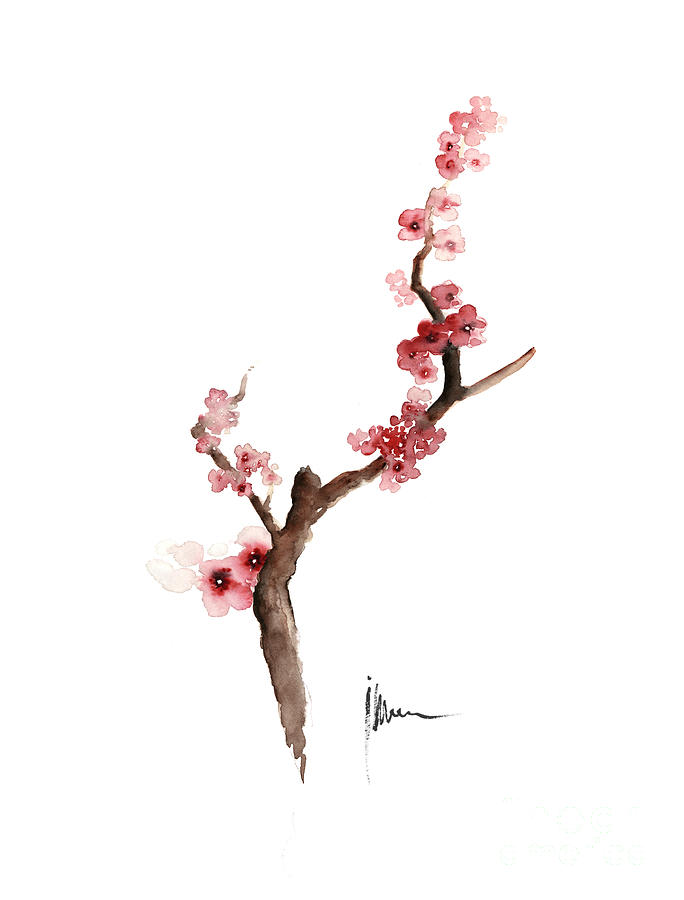This image is a detailed watercolor painting of a single brown branch, likely from a cherry blossom tree, set against a stark white background. The branch, starting from the bottom, curves gently to the right and then more sharply upwards, with a smaller offshoot curving right before the main branch continues ascending left and up. Delicate pink flowers, some of a lighter pink hue and others dark pink with darker pink centers, adorn the left side of the branch and follow its curvature all the way to the top. The petals of the flowers appear fragile and elegant, contributing to the overall delicate aesthetic of the painting. In the lower right corner, there is a small, slightly indiscernible black signature, presumably that of the artist, adding a final touch to this serene and refined composition.